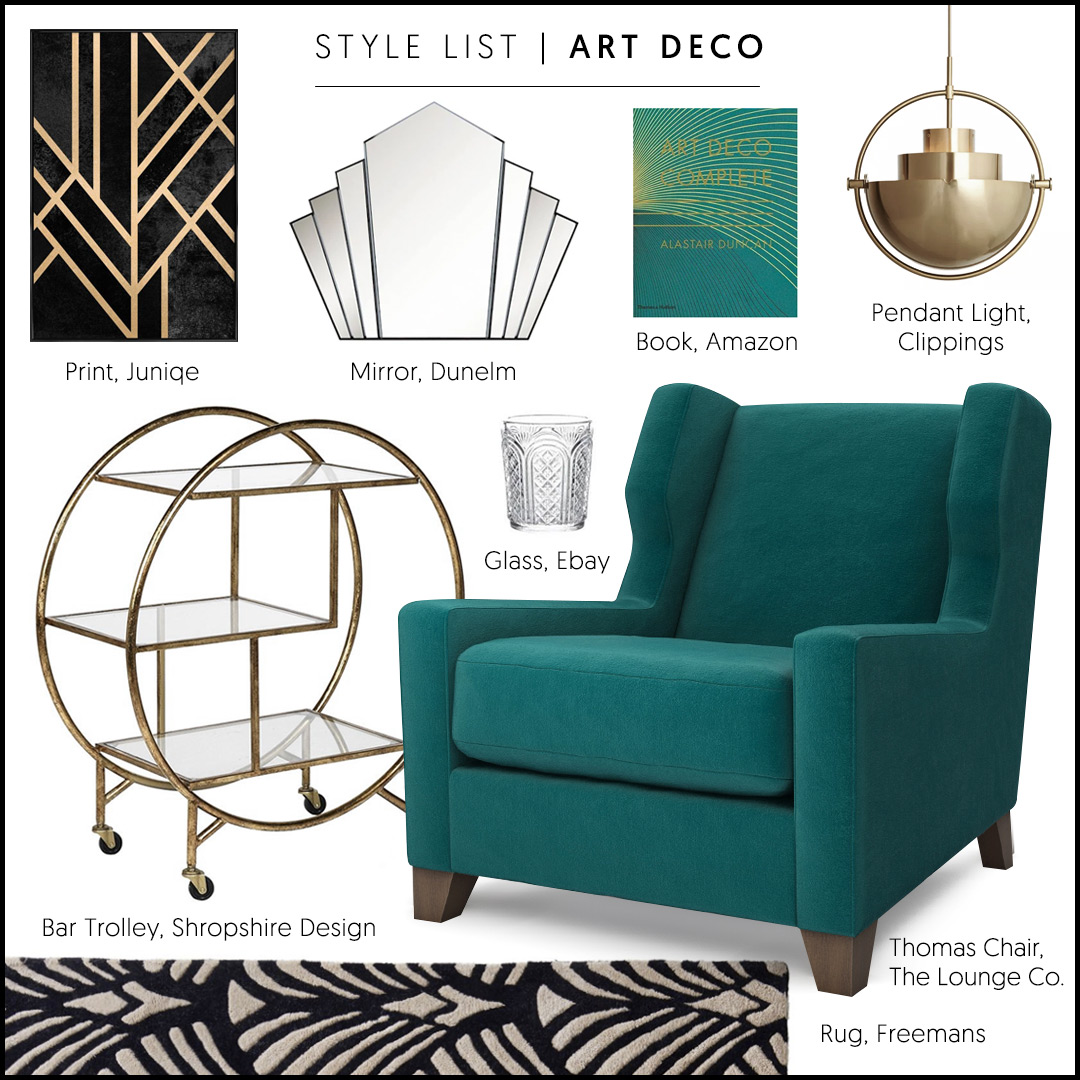The image features a Style List showcasing various Art Deco-inspired furnishings and décor, detailed with a black border framing distinct items. At the top, the caption "Style List - Art Deco" is prominently displayed. 

In the top left, there's a black rectangular print with crisscrossing gold lines, labeled "Print - Genic." To its right, a mirror composed of diagonal sections is titled "Mirror - Dunelm." Next, a green art book with a gold spine is positioned, identified as "Book - Amazon." Adjacent to it is a gold bowl-shaped pendant light, described as "Pendant Light - Clippings." 

At the bottom left, a circular bar trolley with three glass sections and four wheels is labeled "Bar Trolley - Shropshire Design." Above it, a small drinking glass is noted as "Glass - eBay." On the bottom right, a green armchair with brown wooden feet is labeled "Thomas Chair - The Lounge Company." Finally, at the very bottom, a black rug adorned with white angled designs and diamond shapes is marked "Rug - Freeman's."